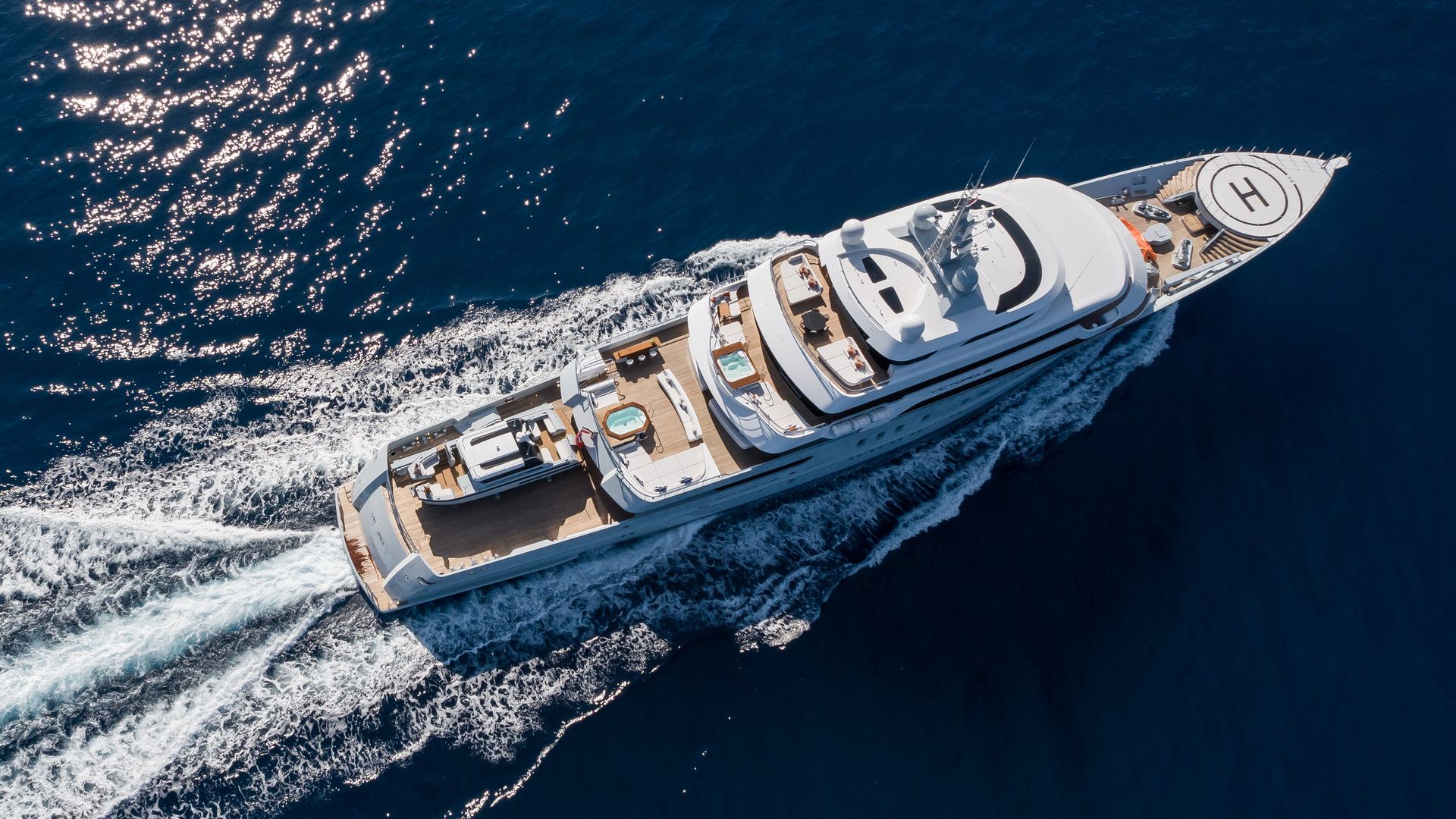This aerial photograph captures a magnificent mega yacht cruising through a vast expanse of ocean, predominantly dark blue with sections of bright blue illuminated by sunlight reflecting off the water's surface in the upper left corner. The yacht, significantly larger than 50 feet—likely closer to 200 feet—slices through the ocean, leaving a trail of white waves and frothy whitewash in its wake, indicating it is moving at a moderate to high speed.

At the bow of the yacht, a circular platform marked with an "H" signifies a helipad, reinforcing the grandeur of the vessel. The yacht features multiple tiers: The topmost deck appears to house an antenna, followed by decks designed for luxurious lounging. The uppermost lounging deck contains tables and seating areas, providing an open space for relaxation. Below this, a deck features a hot tub or possibly a small pool, offering additional leisure amenities. A third level also includes a hot tub with more seating, emphasizing the yacht's opulence.

Towards the stern, the yacht boasts a small secondary boat, likely a motorboat, attached to the rear deck, underpinning the vessel's multifunctional capabilities. The yacht itself is predominantly white with elements of wood-colored detailing, further enhancing its sophisticated appearance. Overall, the yacht's expansive, tiered structure and luxurious features underscore its status as a mega yacht designed for both comfort and leisure on the open sea.